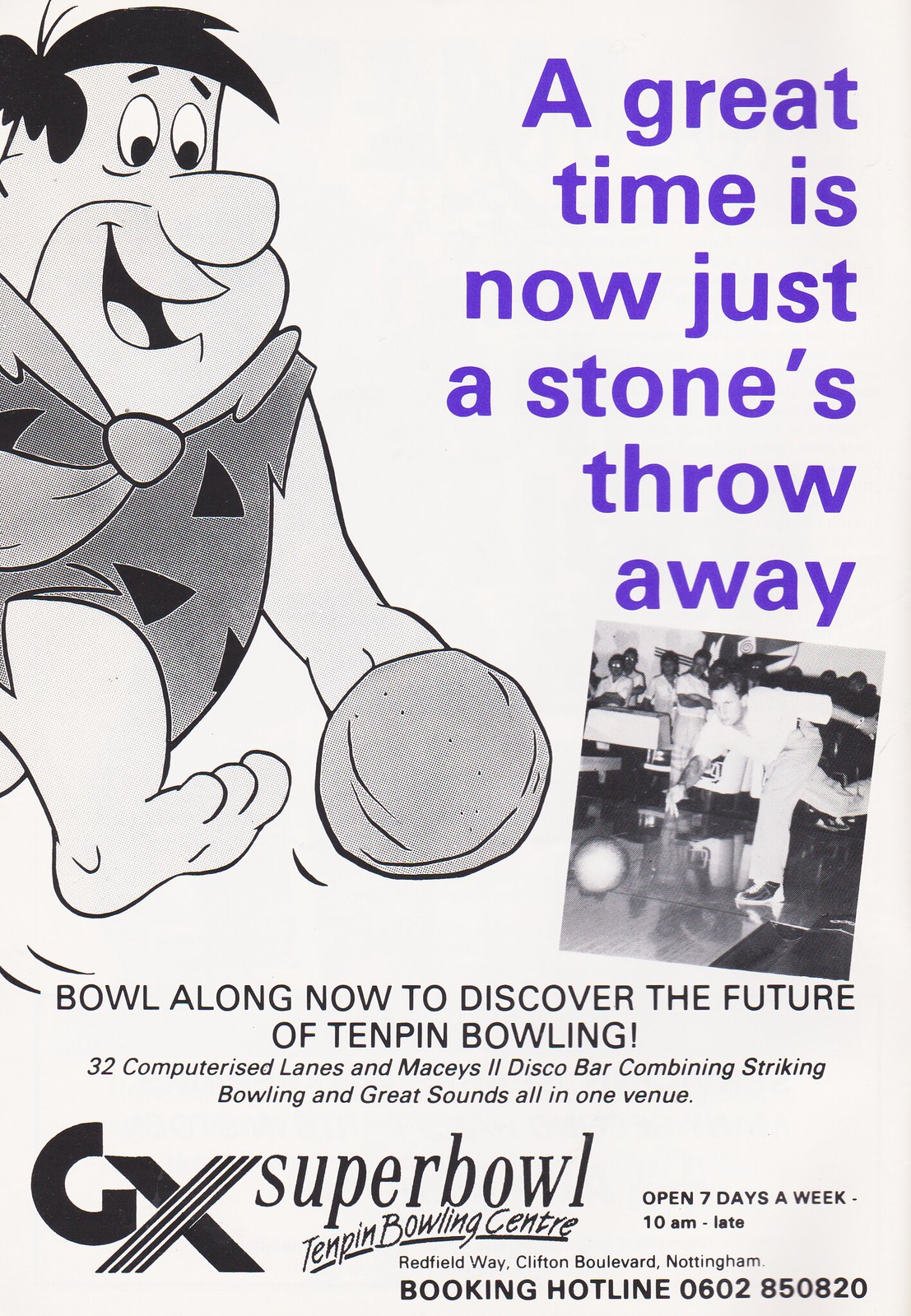This is a detailed full-page advertisement for CX Super Bowl 10-pin Bowling Center. The predominantly black and white flyer features various shades of gray and striking purple text. On the left side, there is a cartoon illustration of Fred Flintstone poised to bowl with a large stone ball. Next to him, a historical black and white photograph depicts a man bowling, giving a nostalgic feel. In bold, purple writing at the top right, it states, "A great time is now just a stone's throw away." Below, the advertisement invites readers to "Bowl along now to discover the future of 10-pin bowling," highlighting the venue's 32 computerized lanes and Macy's 2 disco ball, which combine striking bowling action with fantastic sounds. The large logo at the bottom confirms the location as CX Super Bowl 10-pin Bowling Center, which operates seven days a week from 10 a.m. to late. The address is Redfield Way, Clifton Boulevard, Nottingham, with a booking hotline available at 0602-850-820.